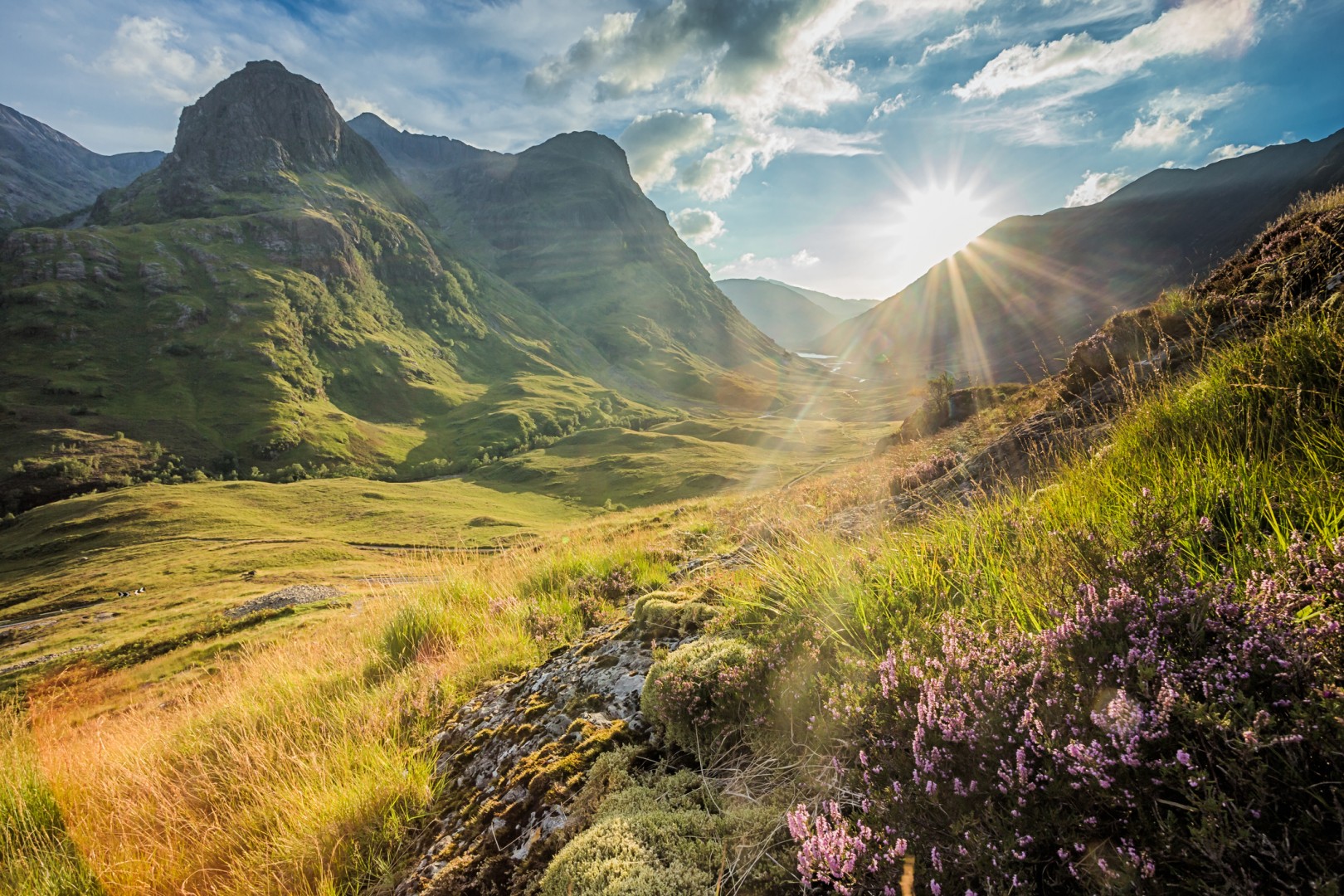The image depicts a breathtaking valley scene under a blue sky dotted with a variety of gray and white clouds, some high-altitude and others puffy but not dense enough to block the sun. Rays of sunlight cascade through the clouds, illuminating the landscape with a serene glow. The valley itself is nestled between two mountain ranges, their peaks covered in green grass and stretching off into the distance. Rolling hills dominate the foreground, with abundant grass shoots blanketing the terrain. On the bottom right, a rock formation rises, adorned with purple wildflowers and shrub-like vegetation. Fields of grass and various plants climb the sides of the mountains, adding to the rich tapestry of the natural setting. This realistic photo, whether slightly edited or AI-generated, captures the tranquil beauty of this daytime landscape with its sun low on the horizon, painting the scene with warmth and light.